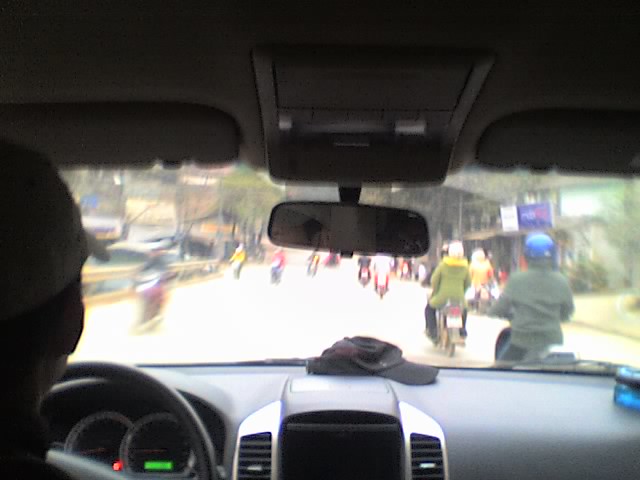This color photograph, taken from the back seat of a left-hand drive car, captures the scene from behind the driver's head, who is wearing a white baseball cap. A black baseball cap lies on the dashboard. The car features a digital dashboard, suggesting it is relatively modern, within the last 20 years. Visible on the gauge cluster are a green rectangle light and a red light. Through the windshield, a bustling street scene unfolds with at least nine motorbikes surrounding the car. Riders are seen with blue and white helmets, while many riders are without helmets. The road is light-colored with a metal guardrail on the left. To the right are various buildings in shades of white and tan, with gray or black roofs. There is a patch of short green grass on the right side of the road, along with a tree. No signs, animals, birds, or flowers are visible in the image.